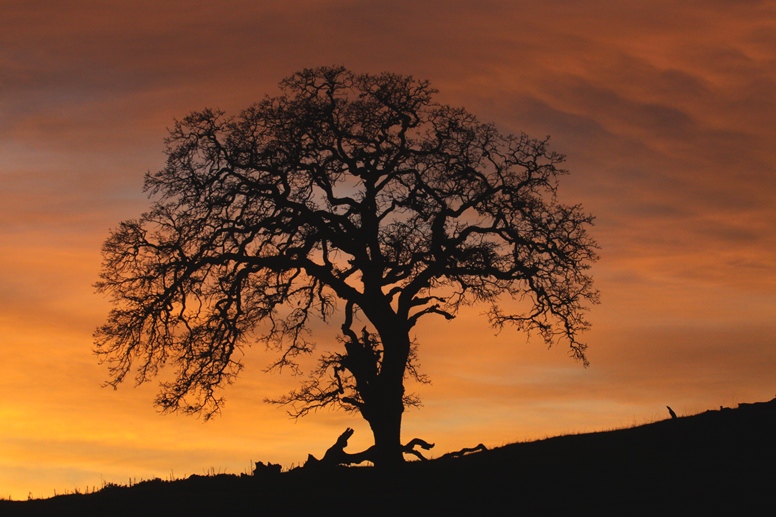The photograph captures a striking scene of an evening sky painted in shades of orange, casting a warm glow over the landscape. A tree, approximately 20 to 30 feet tall, stands prominently in the foreground on a gently sloping hill that rises from the bottom left to the right center edge. The tree itself has a dark, almost black silhouette against the vibrant sky, with its main trunk leaning slightly to the left. The longest branch curves gracefully from the trunk, arcing to the left and extending just below the left center of the frame. Numerous other branches sprout in various directions, with most stretching either straight up or to the right, and the majority of the leaves have fallen, leaving the intricate network of branches exposed. A fallen branch lies behind the tree, adding to the scene's sense of serene decay amidst the glowing backdrop.